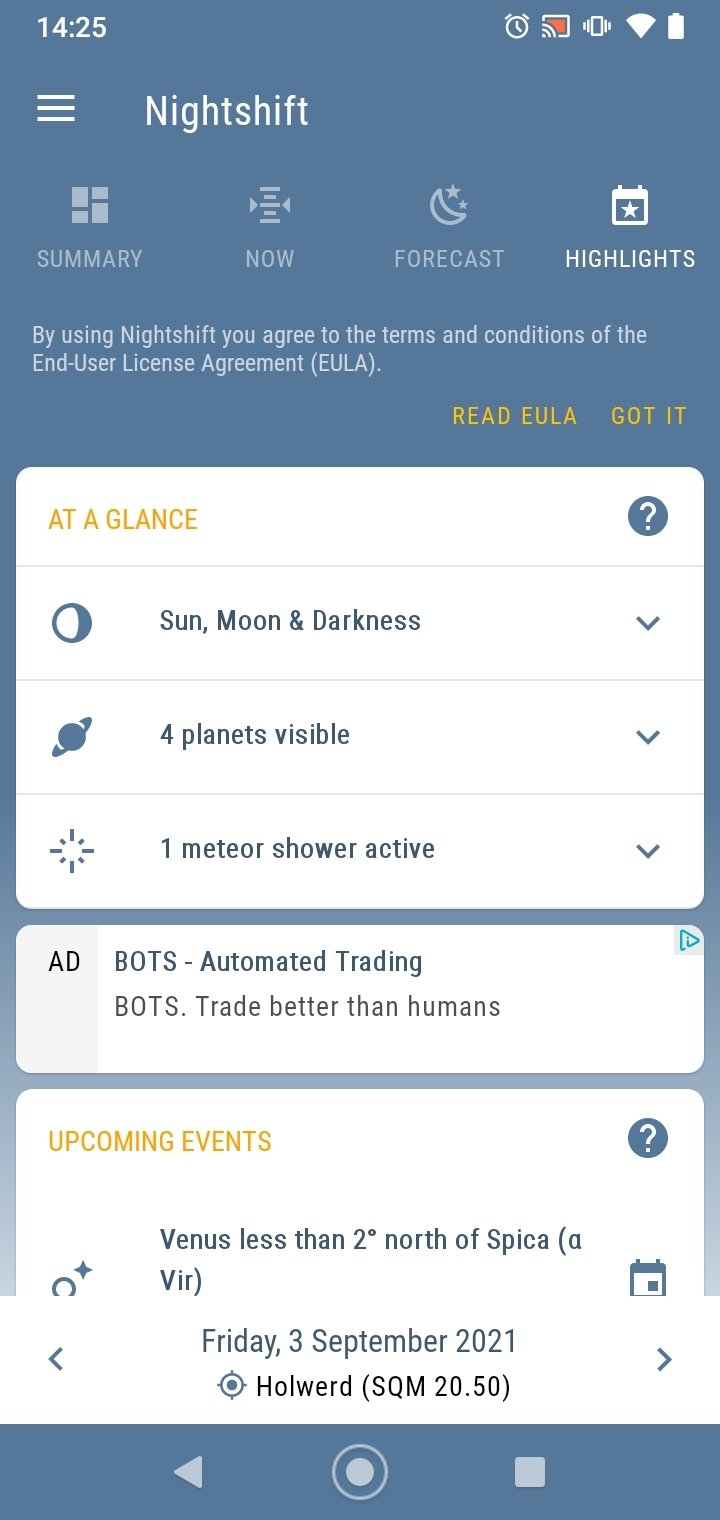This is a detailed screenshot of a smartphone app called "Nightshift." At the top of the screen, the app's title is prominently displayed, followed by a simple text logo. Beneath this, a navigation menu includes several options: Summary, Now, Forecast, and Highlights, each accompanied by small illustrative icons.

Before you start using the app, it prompts you to agree to the user terms and conditions detailed in the End User License Agreement (EULA). There are two buttons to either read the EULA or acknowledge it with a “Got it” option.

The main interface of the app shows four white text fields with softly curved corners:

1. The first field, labeled "At a Glance," has a small question mark icon within a circle on the right, indicating further information is available. Below it, three lines of information are displayed:
   - An icon of a three-quarter moon phase, along with details about the current sun, moon, and darkness status with a dropdown menu.
   - A Saturn-like icon indicating that four planets are visible, also accompanied by a dropdown menu on the right.
   - An icon with rays (possibly representing a meteor shower) suggesting that one meteor shower is active, again with a dropdown menu option.

2. The second text field simply states "Add bots automated trading," followed by a brief promotional tagline: "Bots trade better than humans."

3. The third field highlights "Upcoming Events," detailing that Venus will be less than two degrees north of Spica (Virgo). Accompanying this text are a calendar icon on the right and a planet/star icon on the left.

At the very bottom of the screen are the usual smartphone navigation buttons: Back, Close, and Close All.